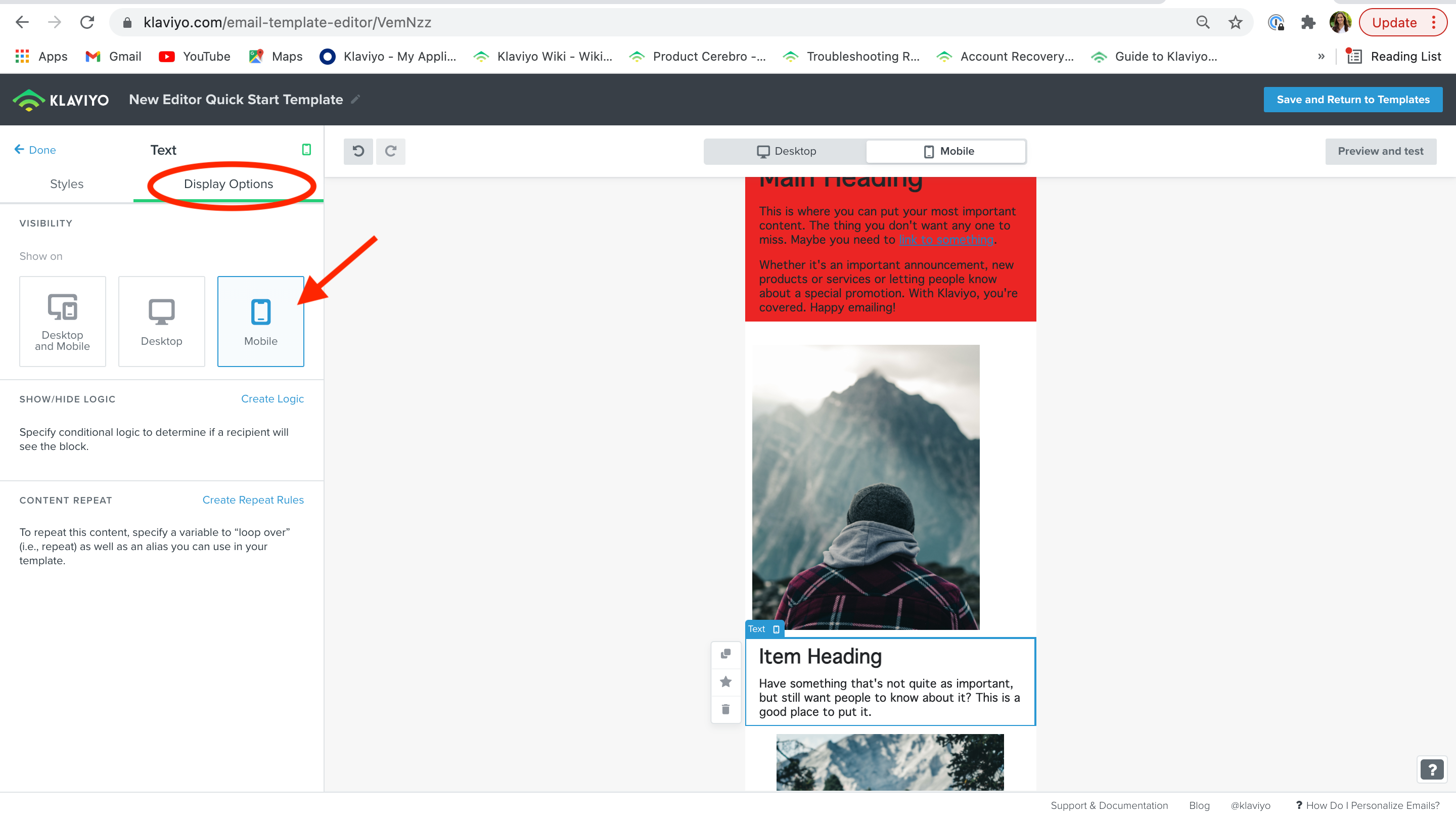The image depicts a screenshot of a website, calveo.com, specifically its new editor thorough the URL calveo.com/editor/vmnzc. The editor features a "Quick Start Template" prominently displayed. 

On the left side of the screen, there are various options available for customization:
- At the top, there is a section labeled "Text" followed by "Style/Display Options."
- Below this section, there are tabs labeled "Desktop" and "Mobile," with a button indicating the selection of the "Mobile" option.
- Further down, there's a section labeled "Show/Hide Logic," which includes a description that reads, "Specify conditional logic to determine if a recipient will see the block."
- Below that, there’s an option titled "Content Repeat," explaining that you can "specify a variable to repeat this content."

At the center of the screen, someone is actively editing a pamphlet or a similar document using the template provided by the editor. The interface seems intuitive, designed to help users effortlessly create and customize email templates or other promotional materials.